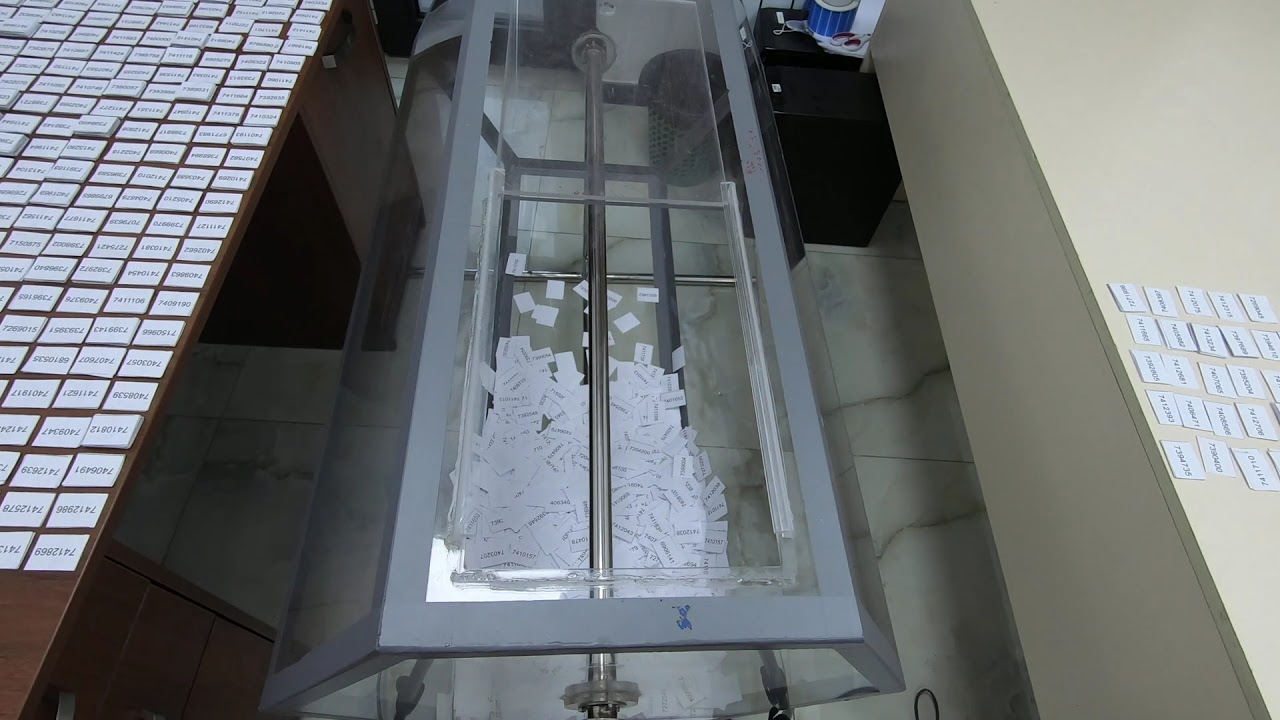The photograph depicts a well-lit indoor scene dominated by numerous small, rectangular labels with numbers printed on them. The left side of the image features a brown wooden table covered with these numbered labels, some in stacks. At the center stands a transparent glass booth containing more of these labels, intersected by metal poles. To the right, a lighter-colored, cream or yellow-gray shelf holds additional labels. The clear and bright image highlights the organized yet chaotic display of numbered slips across various surfaces, with no people present in the scene.